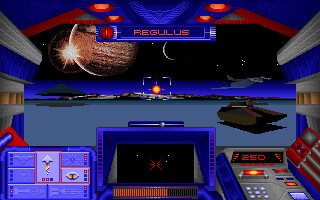The image is a pixelated, landscape-oriented screenshot from an early 2000s video game, possibly on a PC or mobile app. Dominated by shades of blue and red, it presents an interior scene of what appears to be a spaceship or futuristic tank. The focal point is a central rectangle displaying the word "Regulus" in red font on a blue background. In the center of the screen, a crosshair consisting of four blue cornered pieces and a red and yellow circular ball with blue spiky points extends up, down, left, and right, likely indicating a targeting system. 

The lower left corner contains an inventory box, while the right side of the screen features a gray control panel filled with lit-up white and red buttons. Through a clear section of the interface, the exterior scene reveals a smooth, light blue terrain under a blue horizon, with distant pyramids, planets, and moons floating in space. Additionally, a space version of a tank is seen off in the distance, adding to the game's interstellar theme. Above and beyond the control panel, blue-tiled walls with a red border frame the scene, suggesting the player is situated within an enclosed room.